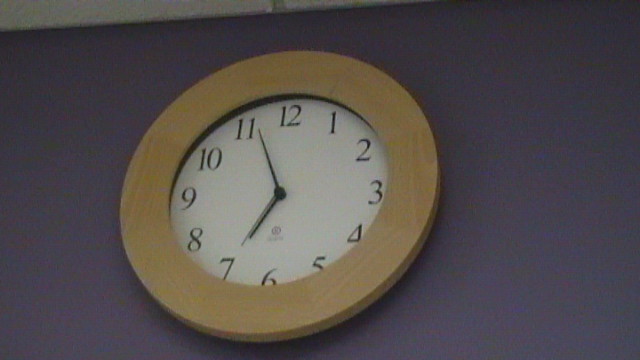The photograph captures an upward view of a wall-mounted clock, taken as if you were standing on the floor and looking up at it. The clock has a thick, light brown wooden frame, approximately three inches wide, which creates a striking contrast against the deep purple wall behind it. The face of the clock is completely white, featuring black numerals from 1 to 12. The hour and minute hands are both black, with the minute hand pointing near the 56-minute mark, while the hour hand is approaching the 7. Additionally, there's a silver second hand aligned with the 7. The manufacturer’s name is inscribed on the clock face, just below the hands’ attachment point, though it is too small to be clearly legible. The image is slightly grainy, particularly on the purple wall, and a glimpse of the white ceiling can be seen at the top of the frame. This scene evokes a classroom or office environment.